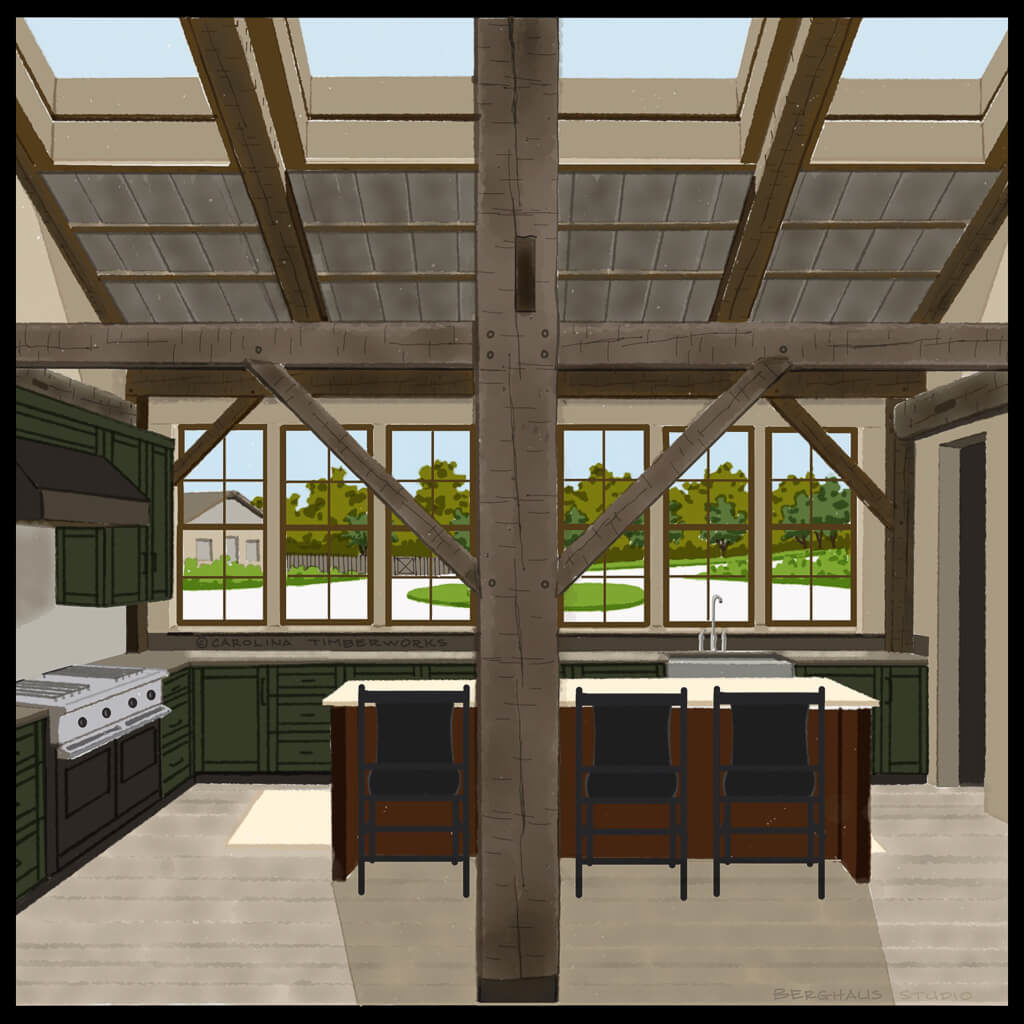This computer-generated image depicts a spacious, open-concept kitchen with a high, slanted ceiling featuring exposed wooden beams that lend a rustic, aged look reminiscent of barn wood. The ceiling is punctuated by four large skylights and is accompanied by gray wooden slats that might slide to cover them. Dominating the room's center is a large, dark brown wooden pillar that extends vertically and is intersected midway by horizontal wooden beams.

The kitchen's layout includes a long counter beneath a series of vertical rectangular windows, each framed in brown. These windows offer a view of a circular driveway bordered by grassy land and an array of trees, with another house visible across the street. Below the windows, green cabinetry complements a white countertop, including a sink positioned along this counter.

To the left is another countertop forming an L shape, housing dual range ovens with a large, black hood vent that has a silver top and black base. This section also features additional green cabinets.

In the middle of the kitchen stands an island with a dark brown wooden base and a white marble top, accompanied by three black chairs neatly pushed under it. The flooring throughout the kitchen appears to be a beige tile, adding a subtle contrast to the bold colors of the cabinetry and countertops.